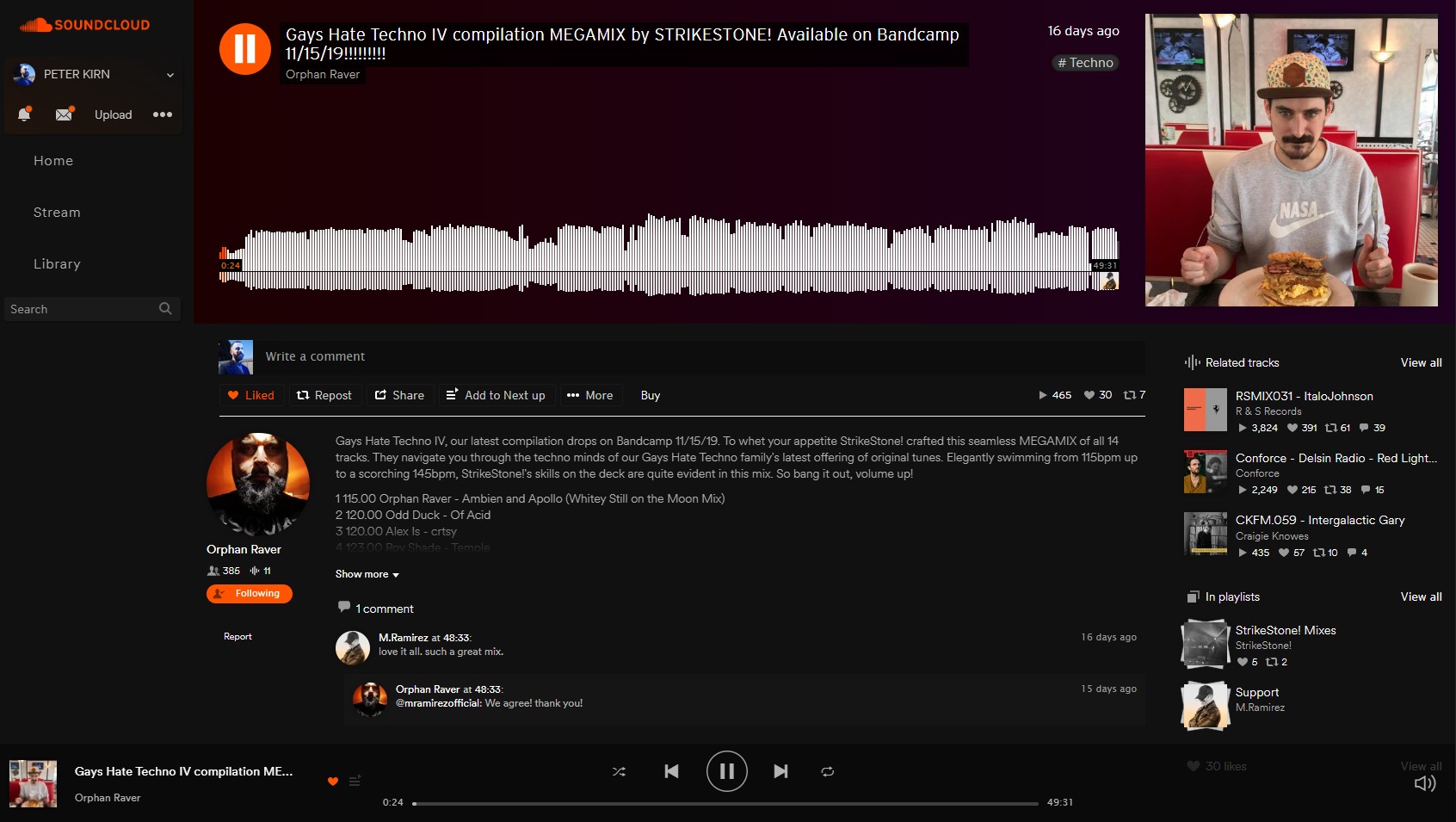The image depicts a SoundCloud music page showcasing the track "Gaze Hate Techno Compilation Megamix" by Strike Stone. The track, which is available on Bandcamp, appears to be paused as indicated by the visible pause button. This megamix includes 14 seamless tracks that navigate listeners through the intricate soundscapes of the latest offering by the Gay Hate Techno family, ranging from a variety of tempos up to a blistering 145 BPM.

Beneath the music player, there is a detailed description of the compilation, mentioning that Strike Stone has crafted an engaging experience designed to captivate one's auditory senses. The page also features the artist Orphan Raver, who has garnered positive feedback from listeners. One comment highlights the enthusiasm for the mix with, "Love it all. Such a great mix."

Additionally, the corner of the image where the sound wave is visible includes a quirky detail: a picture of someone wearing a NASA T-shirt with a Nike logo on it, poised to eat a burger on a plate. This visual adds a personal and informal touch to the overall presentation of the music page.